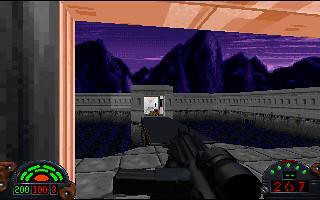This screenshot captures a nostalgic pixel art scene from an older-style video game. At the center of the image, the main character is seen wielding a large black gun, which features a side-mounted sight for precise aiming. The setting is a medieval castle, constructed from gray stone or brick, exuding a formidable atmosphere. Directly ahead, a stone arch frames a glimpse of white light, possibly indicating an approaching opponent that the character is targeting. The background showcases a striking purple sky, suggestive of either dawn or dusk, with silhouetted rock formations or purple mountains lining the horizon, adding an element of dramatic tension to the scene.